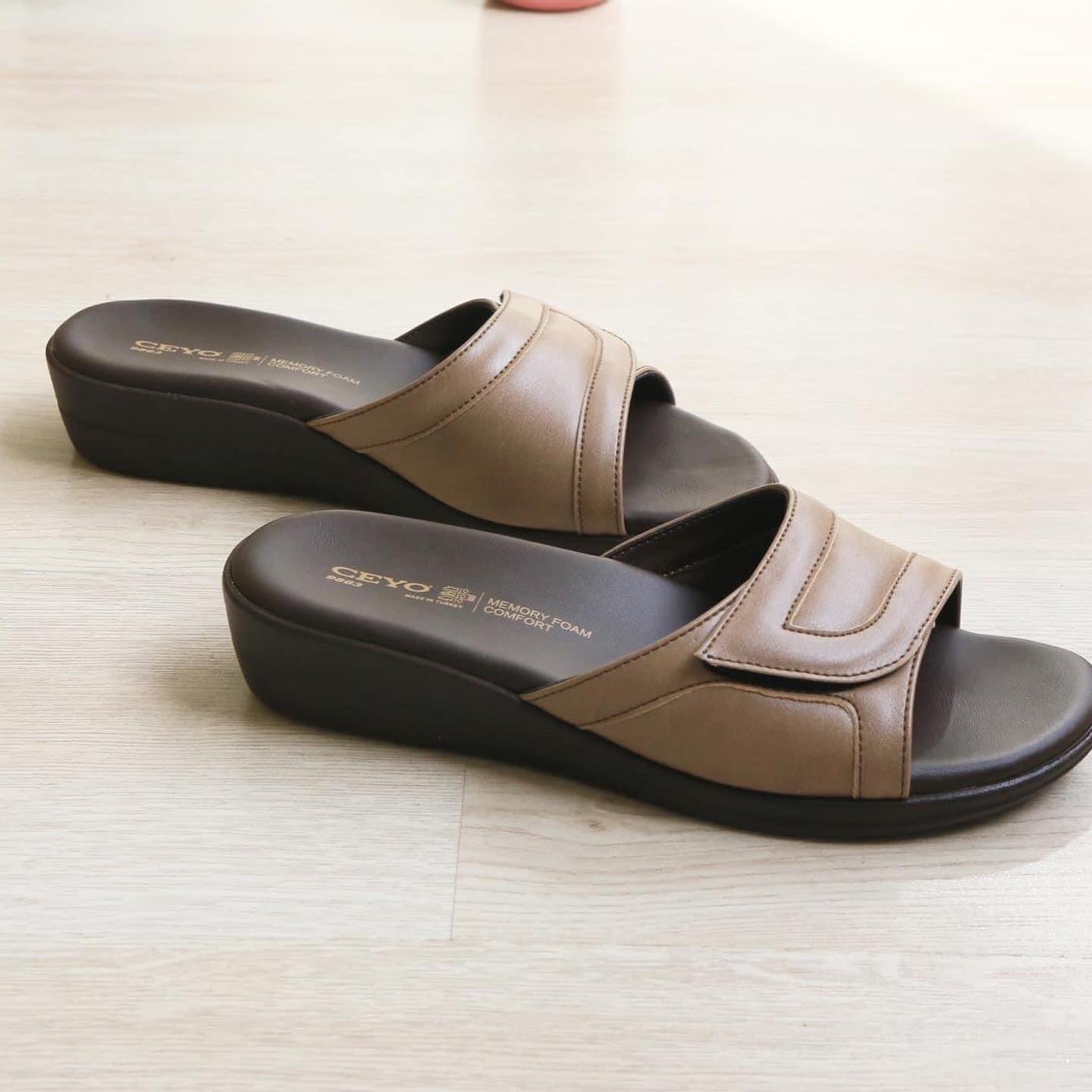In the photograph, a pair of new open-toed sandals are positioned at the center on a very pale, almost off-white, hardwood floor with a horizontally running wood grain. The sandals feature dark brown soles with a slight wedge lift towards the heel. Each sandal is adorned with a wide, lighter brown leather strap that boasts intricate stitching. The straps appear to be held together by velcro, indicating they are in two pieces. The text on the sole of each sandal reads "CEYO Memory Foam Comfort" with some additional smaller, illegible text. The sandals are facing toward the right side of the image, with one slightly ahead of the other, giving the impression they were casually taken off. At the very top center of the square photograph, a thin strip of a red item is visible, though it's unclear what it is. This simple, candid scene suggests a home setting.